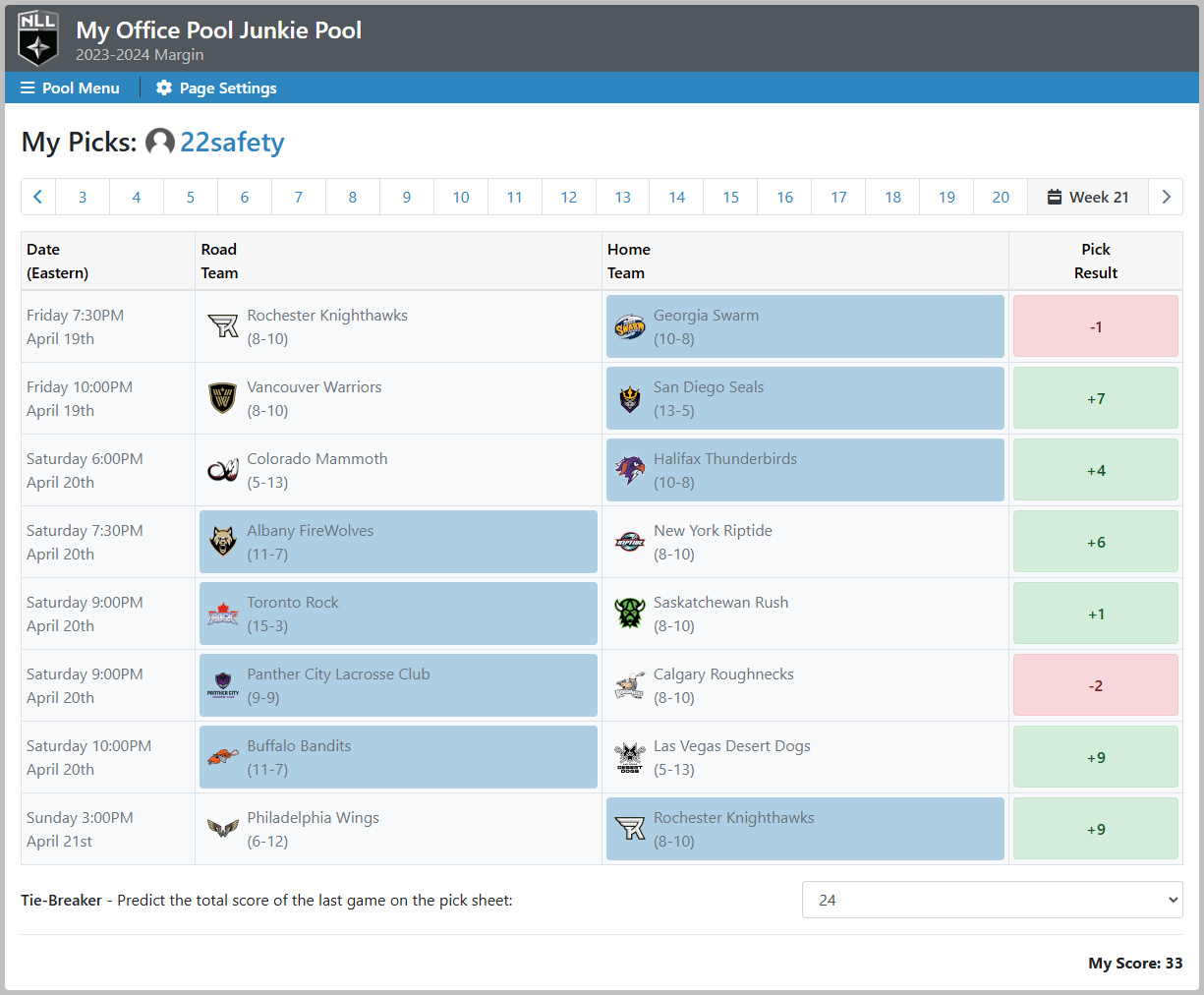This screenshot captures a webpage dedicated to American fantasy football picks. At the upper right corner, prominently displayed is the title "My Picks for Fairway Jake." Just below this heading, it denotes "Week 19." The main section of the page is a chart that categorizes information into four columns labeled as Date, Road Team, Home Team, and Pick Results.

Spanning from January 15th to January 17th, the chart lists various dates, times, and NFL teams, hinting at a range of matchups for that period, though the exact year remains unspecified. The Pick Results column employs a color-coded system to indicate outcomes: green for positive results, red for negative ones, and light blue highlighting certain teams, presumably marking the user's selected picks.

The overall design of the webpage is quite minimalistic, featuring a predominantly white background with light gray text, which could potentially pose legibility issues due to the low contrast. At the bottom right corner, there's a tally of the pick results, summing up the user's performance. The interface exudes simplicity, focused primarily on functionality, and lacks vibrant colors or elaborate design elements.